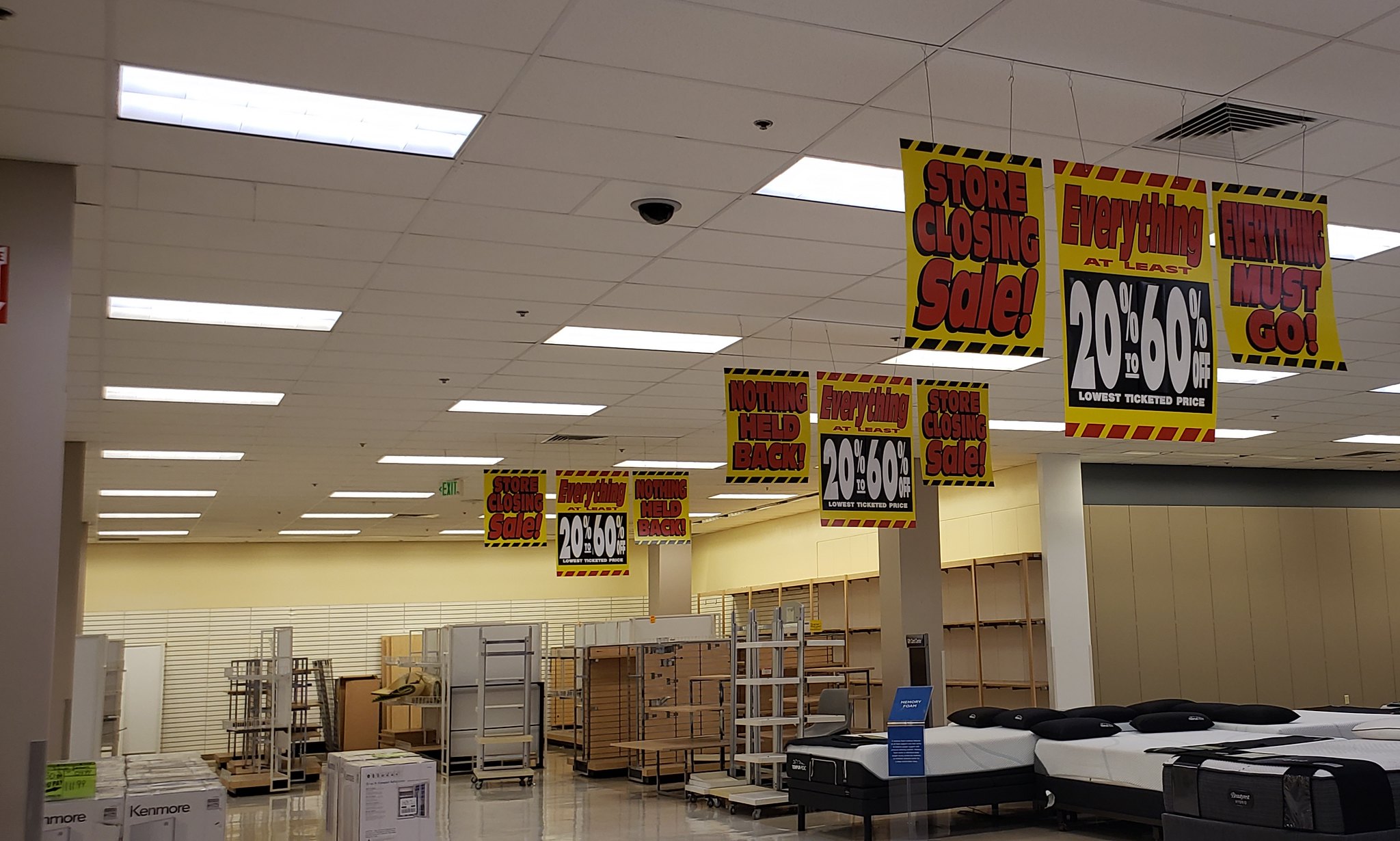This color photograph captures the interior of a large retail store in the midst of a closing sale. The spacious, well-lit room features a greyish-tiled ceiling with rows of large rectangular fluorescent lights. Dangling from the ceiling are multiple yellow banners adorned with big red letters announcing a "Store Closing Sale" and "Everything Must Go." Prominently displayed in the middle of the signs are the words "20% to 60% Off" in white letters on a black rectangle, making the discount unmistakable.

The foreground and midsection of the image reveal numerous empty shelves and largely vacant displays, indicating that the stock has been significantly depleted. Scattered throughout are various items, such as some white and blue boxes in the lower left-hand corner and a small blue rectangular sign with unreadable white text in front of what appear to be several horizontal tables or bins with black bottoms and white tops. 

On the right side of the image, there are some brown-framed beds with white sheets and brown pillowcases, and further back, a series of shelves possibly featuring a few office chairs or Kenmore appliances. Despite these scattered items, the overall impression is that the store is nearly empty, reflecting the final stages of its clearance. The absence of people and windows contributes to a stark, antiseptic atmosphere lit solely by the fluorescent lights, which leaves the exact time of day indeterminate.